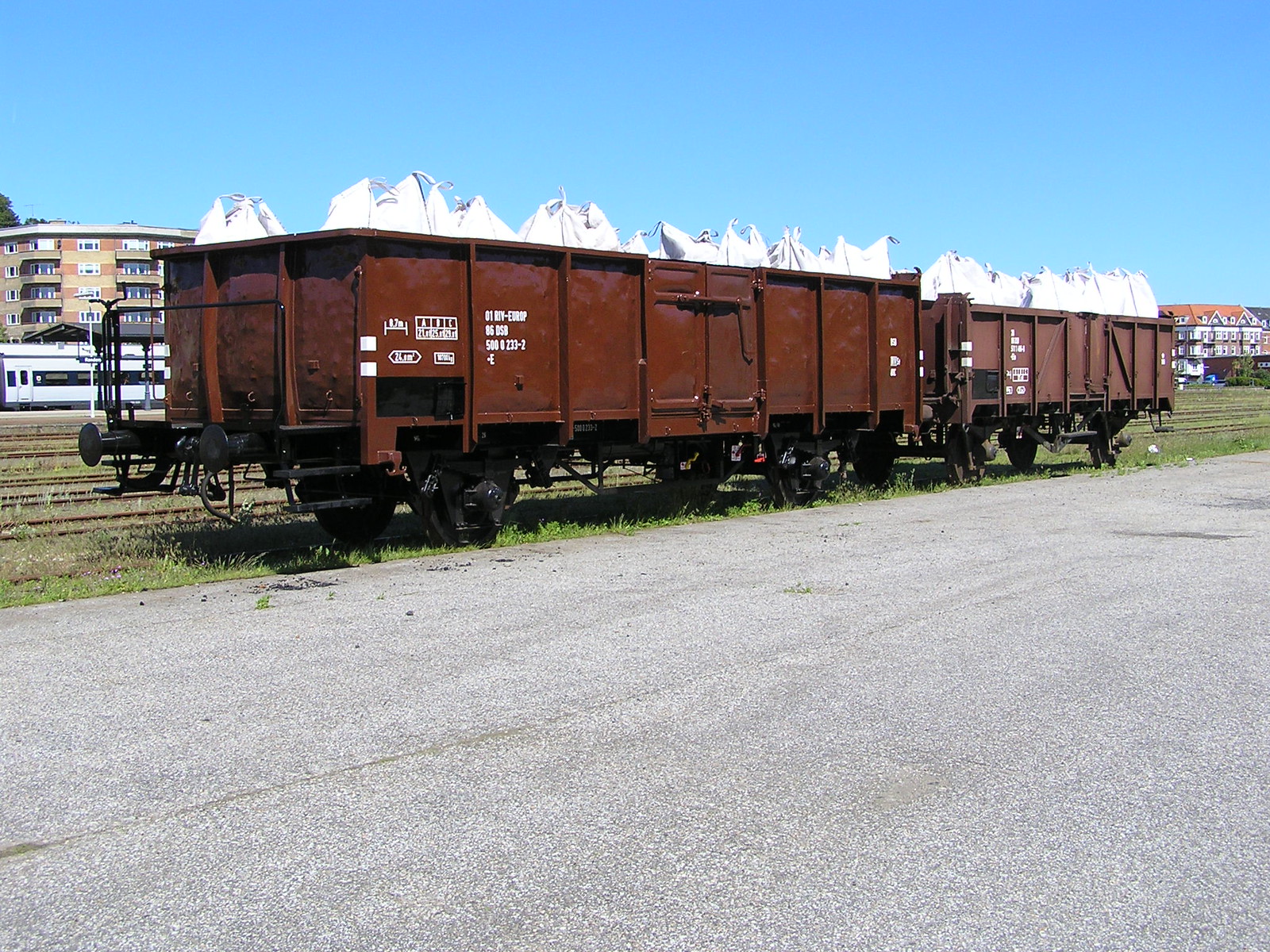This photograph showcases two rectangular, open-top railroad boxcars, one dark brown and the other light brown, resting on a grassy area adjacent to rusted train tracks. The boxcars, designed to run on tracks with their steel wheels, are currently stationary and filled with large white bags. These bags, bulging and tied at the top, appear to be filled with contents of significant size, resembling small tents. The boxcars sit near a gray pavement, with three sets of railroad tracks visible behind them. In the background, apartment complexes mark a near-city environment, framing the scene and adding to the juxtaposition of urban and industrial elements.